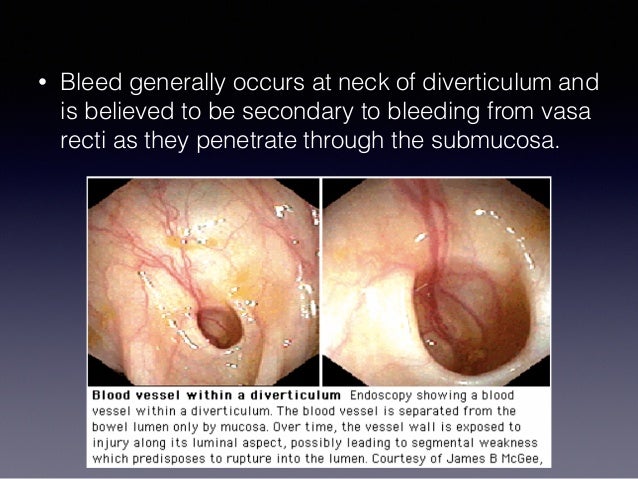The image resembles a slide from a medical presentation. It features a dark blue border with white text at the top that reads, "Bleed generally occurs at the neck of the diverticulum and is believed to be secondary to bleeding from vasa recti as they penetrate through the submucosa." Below the text are two photographs side by side, each depicting a blood vessel within a diverticulum. The left photograph shows the blood vessel with a small hole, while the right photograph displays a larger hole. The area is described as being within the human body, likely observed via endoscopy. The accompanying text beneath the images in black on a white background explains that the blood vessel is separated from the bowel lumen only by mucosa. Over time, this separation exposes the vessel wall to injury, weakening it and potentially leading to rupture into the lumen. The medical content is credited to James B. McGee. The colors in the slide include shades of blue, black, white, gray, red, and tan, suggesting a visually descriptive focus on the anatomical details presented. The positioning of text and images is methodical, indicative of an educational medical setting.